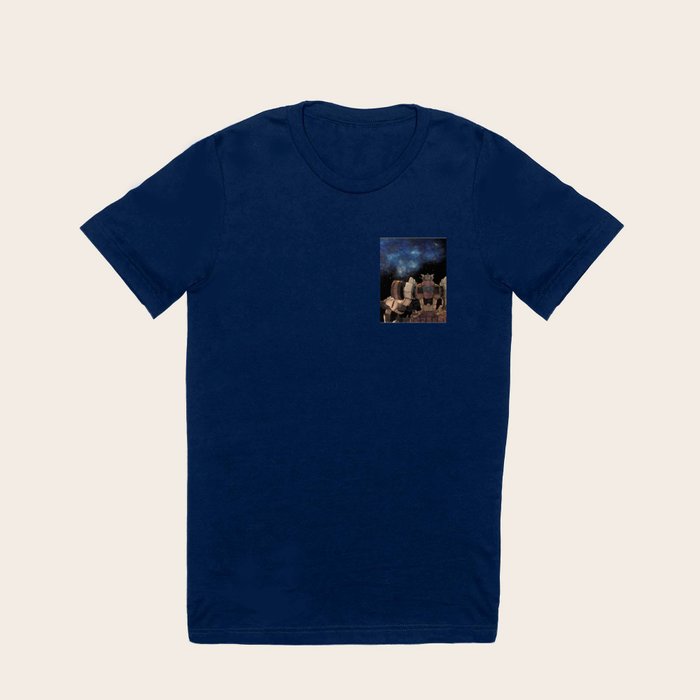The image shows a dark navy blue, short-sleeved t-shirt with a round neckline. On the upper left chest area of the shirt, over where the heart would be, there is a small, square image. The image appears to depict a galaxy-like skyline with swirling blue colors, resembling stars or an ocean under a night sky. This scene is enveloped by black clouds, adding to its surreal and mysterious appearance. Among the clouds, there's a figure that looks like a stone or brick person with distinct features—two eyes and a mouth—rendered in a dark brick red color. Next to this figure, another stone-like object is partially visible, though its exact form is difficult to discern.